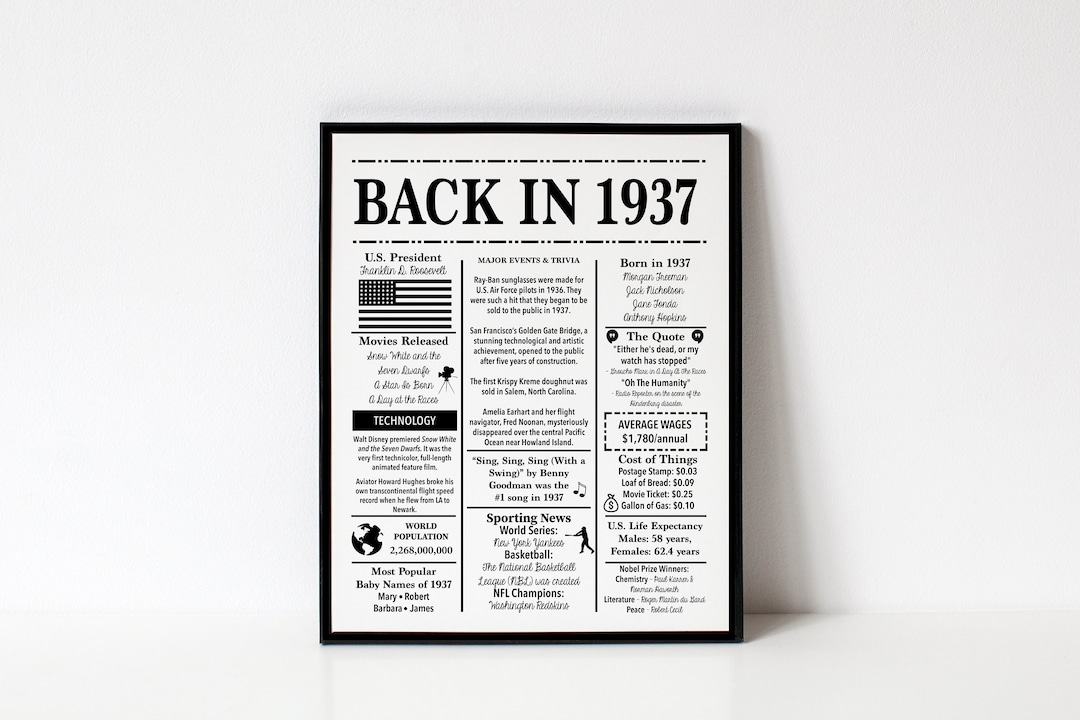This image depicts a framed plaque with a white background, propped against a white wall, casting a shadow to the right. The plaque appears to be a piece of paper mounted on foam core, featuring a black round outline and some decorative elements across the top and bottom. Between these decorative lines, the bold, serif-typed words "Back in 1937" are prominently displayed. The content is organized into three columns filled with various facts and trivia from the year 1937. The left column includes an American flag, a bar with reverse type, and a globe. The center column features a tiny cartoon of a baseball batter, mentions of the US president at the time, Franklin D. Roosevelt, sporting news from the World Series and NFL, and a list of movies released in 1937. The right column highlights details such as most popular baby names, major events and trivia, average wages ($1,780 annually), cost of living, and US life expectancy. Despite the plurality of text on the plaque being too small to read, the overall impression is of a commemorative piece that encapsulates notable historical and cultural highlights from 1937, making it likely intended as a nostalgic gift.